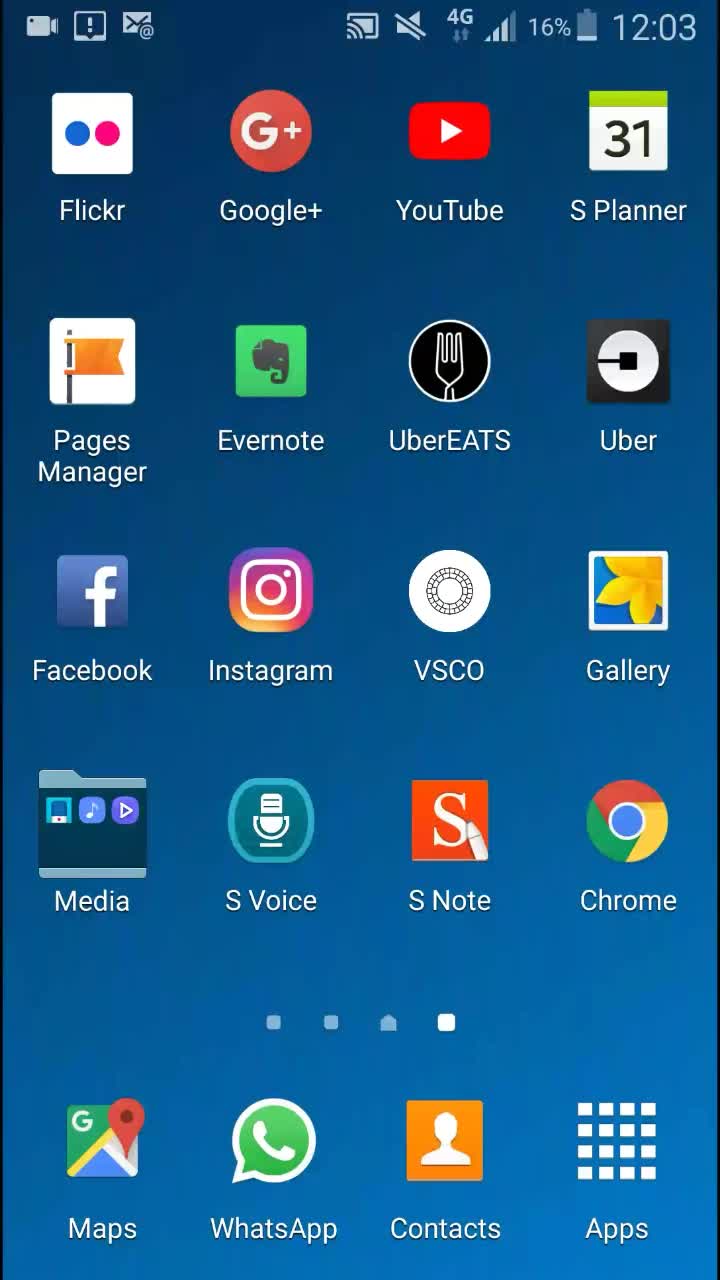The screenshot displays a smartphone home screen featuring an array of application icons arranged in a grid against a deep royal blue background. Positioned at the top of the screen, the status bar shows a light blue design element indicating the battery is at 16% charge, alongside the time, which is 12:03. 

The first row of apps includes: 
- Flickr (spelled out as F-L-I-C-K-R) 
- Google+ 
- YouTube 
- S Planner (which displays the number 31).

In the second row, the apps listed are: 
- Pages Manager
- Evernote
- Uber Eats
- Uber.

The third row consists of: 
- Facebook 
- Instagram 
- VSCO 
- Gallery.

On the fourth row, the icons shown are: 
- Media 
- S Voice 
- S Note 
- Chrome.

Finally, in the fifth row, the applications featured are: 
- Maps 
- WhatsApp 
- Contacts
- an icon labeled "Apps".

The overall color palette is vibrant and diverse, with little blue icons against the predominantly blue background, and app icons showcasing a spectrum of colors including orange, green, red, black, and white. Each app icon adds to the multi-colored visual appeal of the screen.